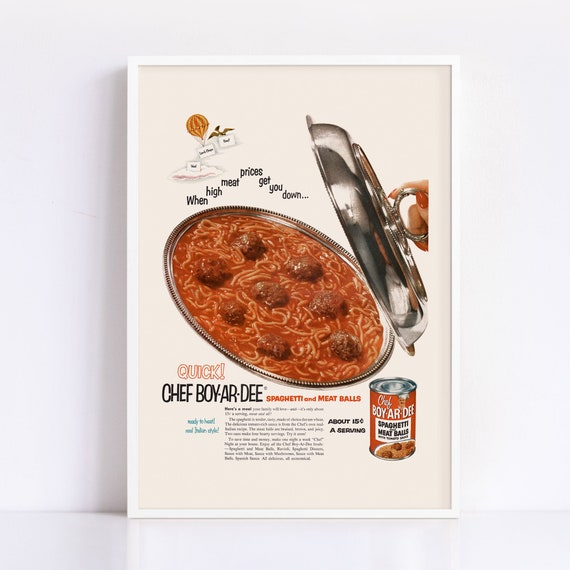This framed advertisement from Chef Boyardee, likely from the 70s or 80s, captivates with its vibrant imagery and nostalgic appeal. The focal point is a large silver dish filled with spaghetti and meatballs, garnished in a rich red sauce. The dish, which prominently showcases the meatballs, is being unveiled by a woman's hand adorned with red nail polish, as she lifts the lid. Bold text at the top reads, "When high meat prices get you down," emphasizing the affordability of Chef Boyardee. The dish, set against a white frame, features a can of Chef Boyardee spaghetti and meatballs in the lower right corner, highlighted with the slogan, "Quick! Chef Boyardee Spaghetti and Meatballs." The ad also includes a small, albeit unreadable, blurb extolling the convenience and appeal of the product, enhancing its eye-catching and appetizing presentation.